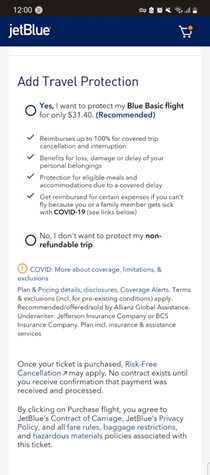This image is a detailed screenshot of a JetBlue booking page displayed on a cell phone. At the top, there's a thin black banner showing the time "12:00" in white text, accompanied by various status icons on the right side: Wi-Fi signal, cellular signal, alarm, muted volume, and a shopping cart.

Below this, a blue banner with a yellow-orange circle holds the JetBlue logo, with a capitalized "B". The main content features a white background with a prominent heading that reads "Add Travel Protection." 

Beneath this heading, there are two radio button options: 
1. A circle labeled "Yes, I want to protect my Blue Basic flight for only $31.40 (Recommended)," in blue text. 
2. Another circle labeled "No, I don't want to protect my non-refundable trip."

Between these options, four check marks detail what the travel protection covers, emphasizing reimbursement benefits. An orange circle with an exclamation point highlights important information related to COVID-19. 

Lower on the screen, the page provides additional information about the ticket being purchased and mentions a risk-free cancellation policy.